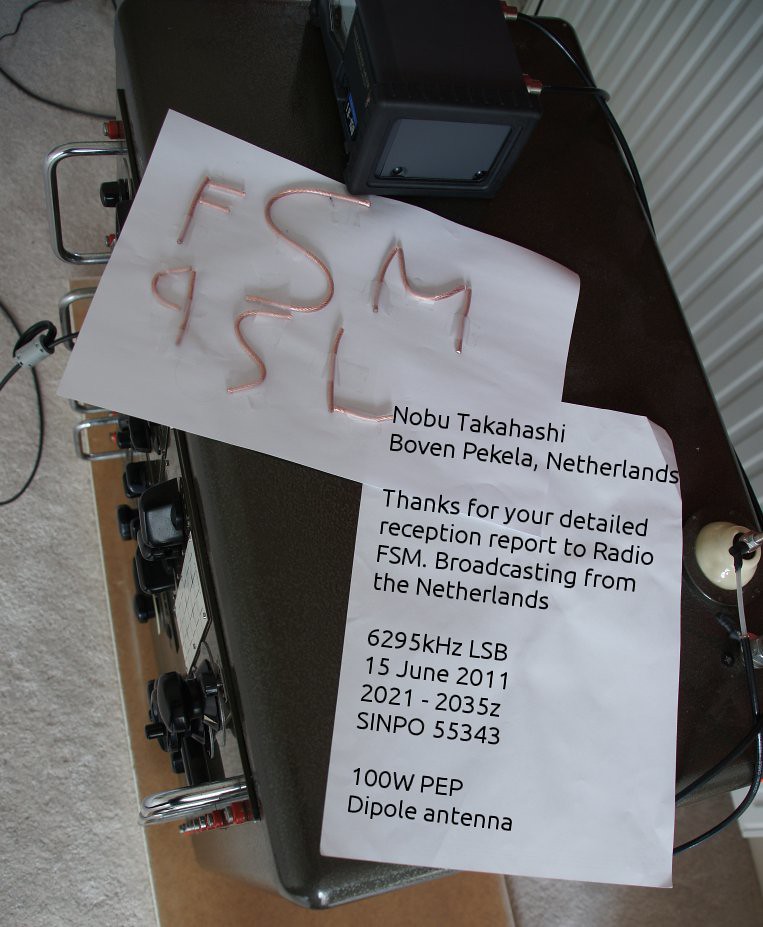This photo depicts two pieces of white paper placed on top of what appears to be radio broadcasting equipment. The equipment is a large, boxy machine adorned with numerous dials, switches, and chrome vertical handles. Various plugs and cords extend from the machine, and a smaller black device with cords rests on top of it. The scene is set on a table with a beige or eggshell white carpet and against a white corrugated wall, suggesting the photo was taken indoors under natural light during the daytime.

One piece of paper prominently features the letters "FSMqsSL" formed out of copper wire and taped to its surface. The other piece of paper contains printed black text reading: "Nobu Takahashi, Boven Pekela, Netherlands. Thank you for your detailed reception report to Radio FSM broadcasting from the Netherlands, 6295 kHz LSB, 15 June 2011, 2021-2035Z, SINPO 55343, 100 watt PEP, dipole antenna." The equipment and papers combined suggest a documentation or acknowledgment related to shortwave radio broadcasting.